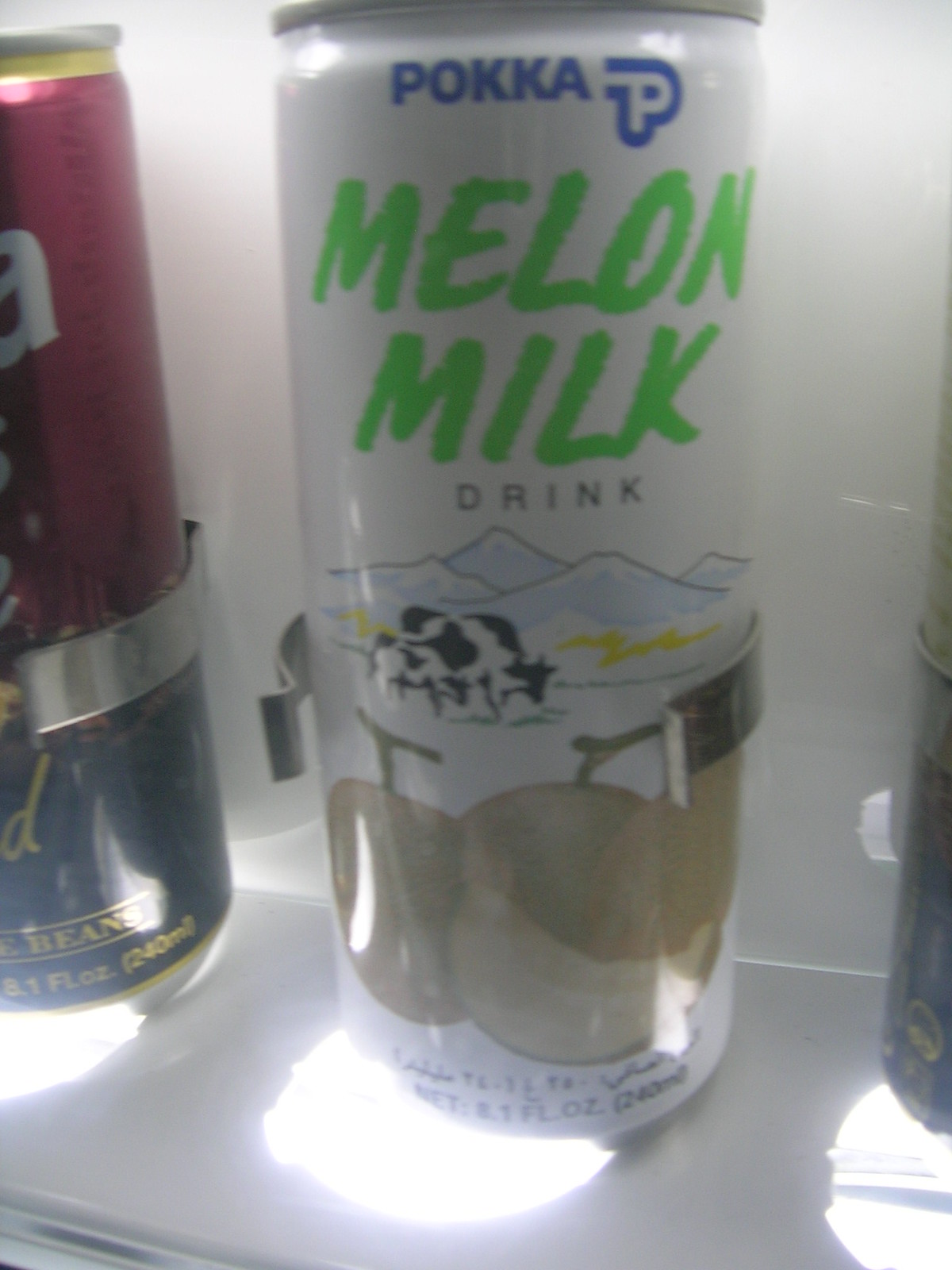The image features a close-up of an aluminum can labeled "Melon Milk," branded by Poca. The can, standing prominently in a well-lit display, showcases vibrant and detailed graphics. It has blue lettering at the top, spelling out "Poca," and beneath it, in green text, it reads "Melon Milk Drink." The illustration on the can includes a picturesque mountain range with two grazing cows—a girl cow and a baby cow—in front, reinforcing a pastoral, natural setting. Additionally, there are images of two brown fruits with stems towards the bottom of the can. The whole scene is illuminated by three lights, highlighting the can’s design, colors, and intricate details, making it the focal point against the minimal background of the display.